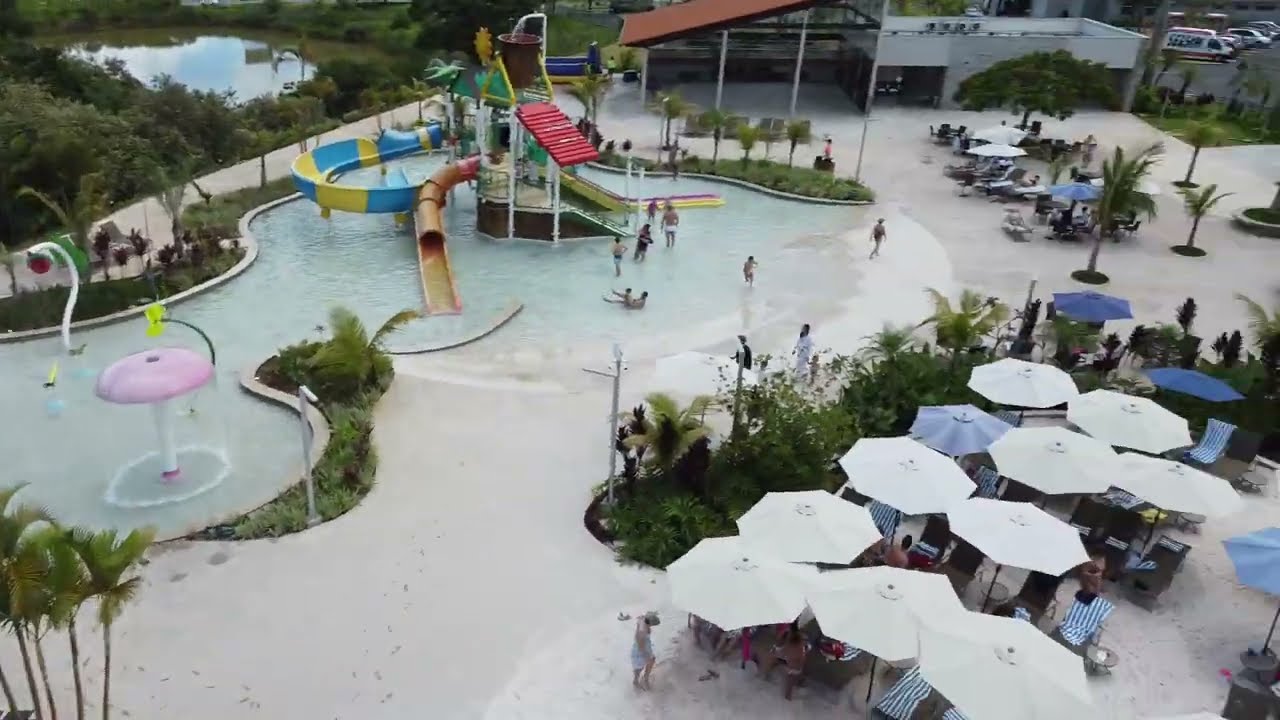This is a detailed aerial color photograph, taken from a drone, showcasing an outdoor water park in landscape orientation under overcast skies. Prominently featured on the left side are two curved pools; the central one houses blue and yellow striped circular slides, a brown tunnel slide, and a purple and yellow slide, along with a pink mushroom-shaped sprinkler structure in the bottom left pool. The image captures bustling activity with people enjoying the water attractions. Surrounding the pools, on the bottom right, is a seating area with various white, light blue, and blue umbrellas shading patio tables, where people sit and children play nearby. The park is lush with palm trees, bushes, and plants, offering a tropical feel. Adjacent to the park is a gray stone cement building, likely the main entrance, and a small pond surrounded by green grass and trees. In the upper right-hand corner, a parking lot with cars is visible beyond the park, with a curved sidewalk encircling the entire area, enhancing the realism and representational style of the scene.